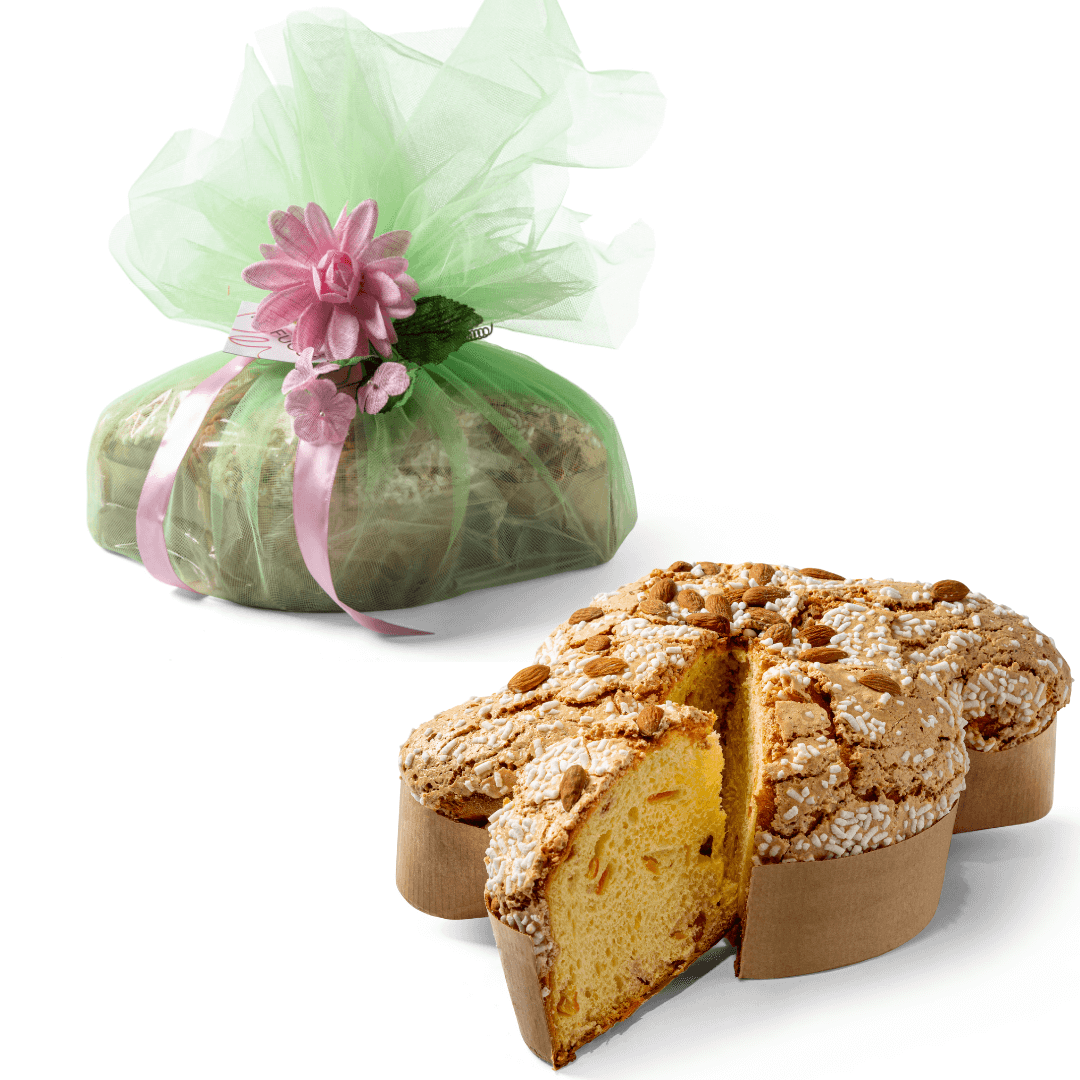In this picture, we see two closely related items that appear to be a type of cake. In the top left part of the image, there is a heart-shaped cake wrapped in a light green wrapper, which is adorned with pink ribbons and a pink flower on top. The wrap material is thin and slightly see-through, resembling a bridal veil, allowing a glimpse of what’s inside. A little label is attached to the side of the wrap.

Below the wrapped cake, there is an unwrapped heart-shaped cake, brown in color with a slightly cracked surface. The top of this cake is decorated with sesame seeds, slivers of almonds, and what appears to be small, rice-like sprinkles scattered throughout. A piece of the cake has been cut out, revealing a light yellow interior speckled with various seeds. The unwrapped cake seems to be encased in a brown, uniquely shaped paper that features curved and interwoven patterns.